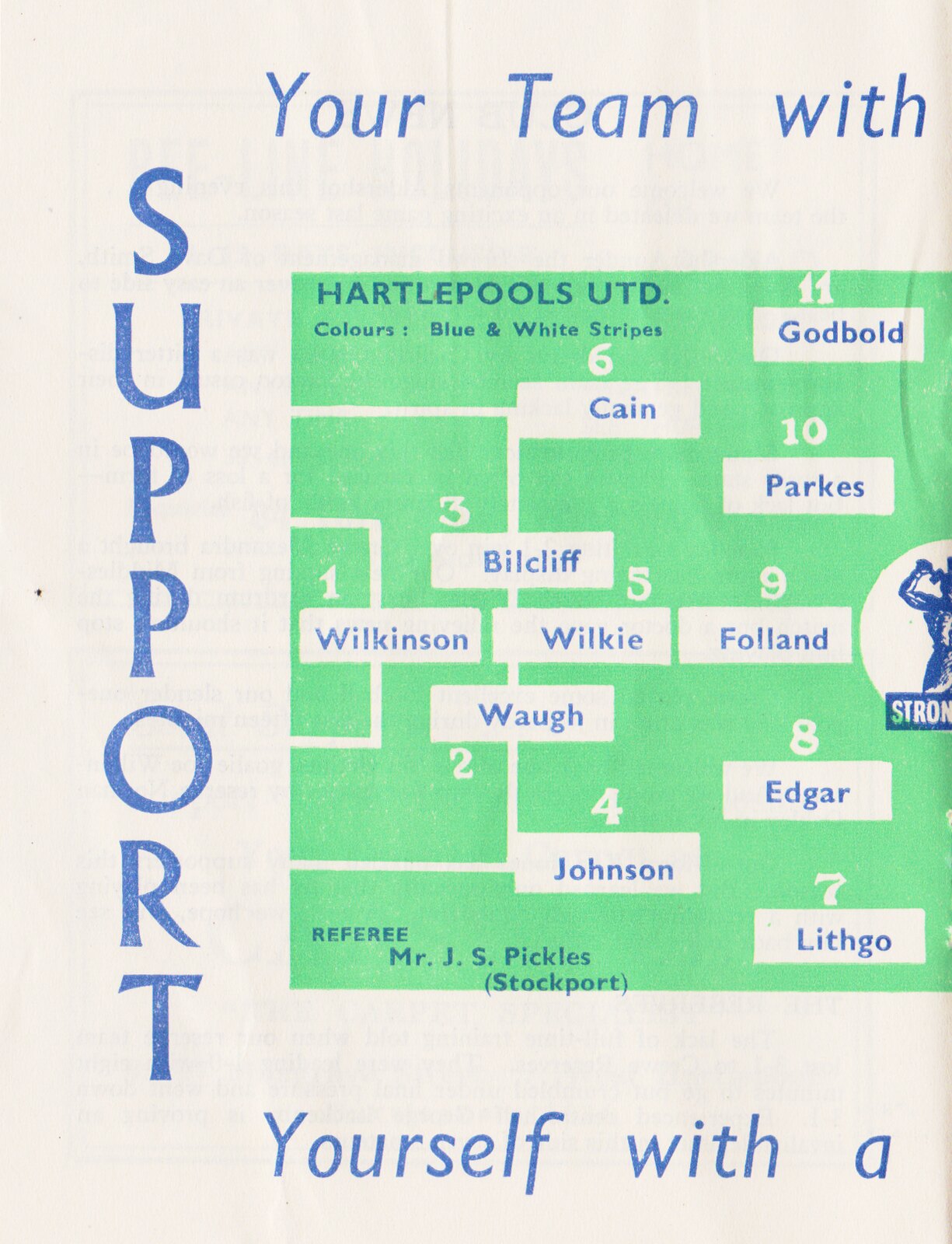The image depicts a folded poster in portrait view, likely cut off because of the way it's positioned. The top of the poster prominently features the partially visible text "your team with" in blue, with "support" running vertically down the left side and the partially readable "yourself with a" at the bottom. The center of the poster, set against a green background, showcases a football (soccer) team's formation on a field.

The formation reveals players' numbers and names, presented in blue text on a white background. Specifically, the names and numbers are as follows: 1 Wilkinson (goalkeeper), 2 Wall, 3 Bilcliffe, 4 Johnson, 5 Wilkie, 6 Kane, 7 Lithgow, 8 Edgar, 9 Poland, 10 Parks, and 11 Godbold. The upper section of this central formation area also contains the text "Hartlepool United, colors blue and white stripes," indicating the team and their colors. Despite the partial view, the image is a detailed depiction of the football team's lineup and structure, laid out in a traditional sports bracket style.